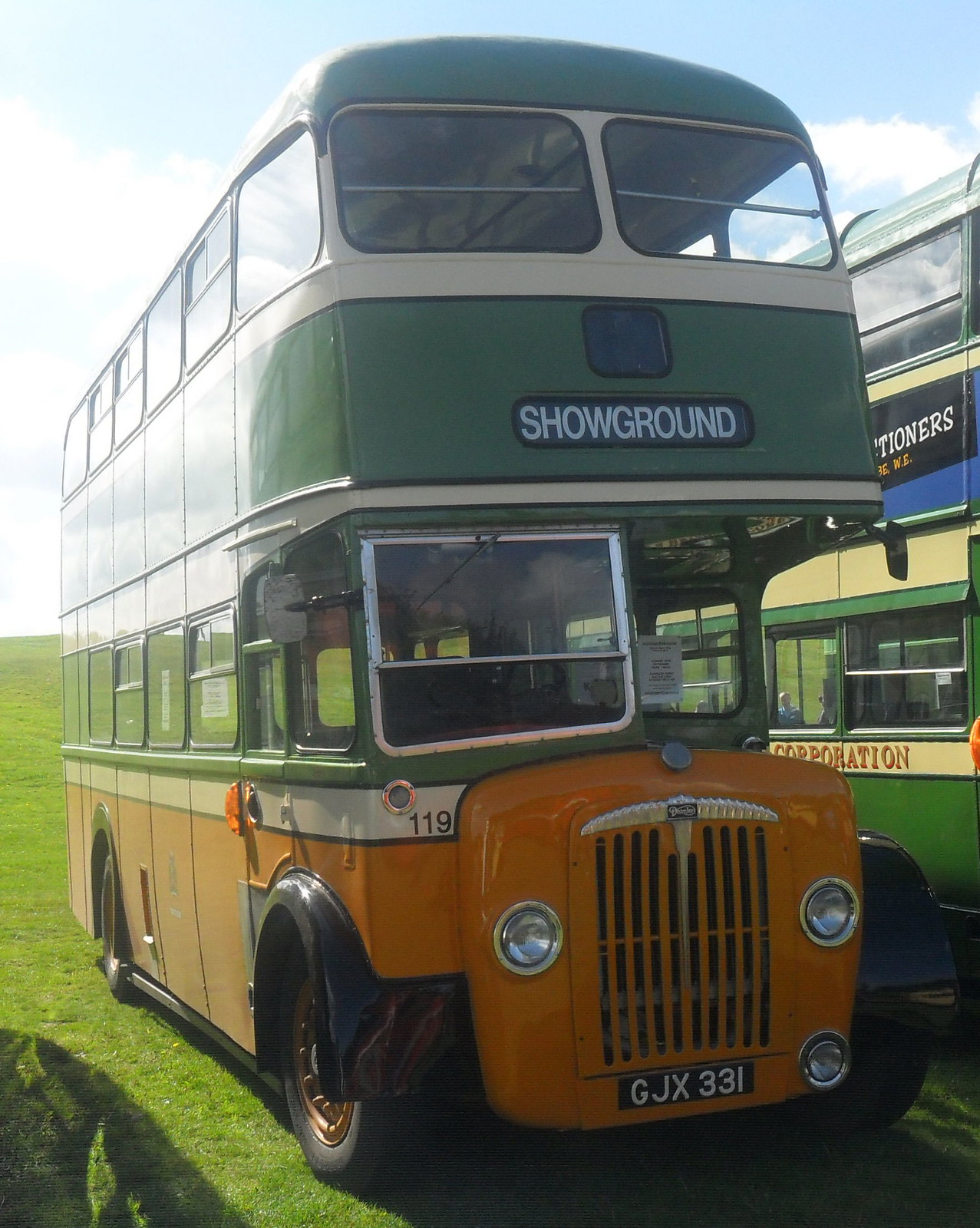A well-maintained, old double-decker bus is prominently featured in a grassy field. The bus, primarily painted green with detailed white accents, including a stripe, has an orange lower section that extends around the front. The front boasts a small windshield and windows spanning both levels, framed by black around the wheels. It bears a black license plate, GJX331, and a sign between the decks displaying "Show Ground" in white font. On the left side, under the driver's window, the number 119 is visible. A second bus, partially obscured, stands to the right, appearing to be a different model, also adding to the scene's vintage charm. The buses are set against the backdrop of vibrant, green grass, enhancing the nostalgic atmosphere.